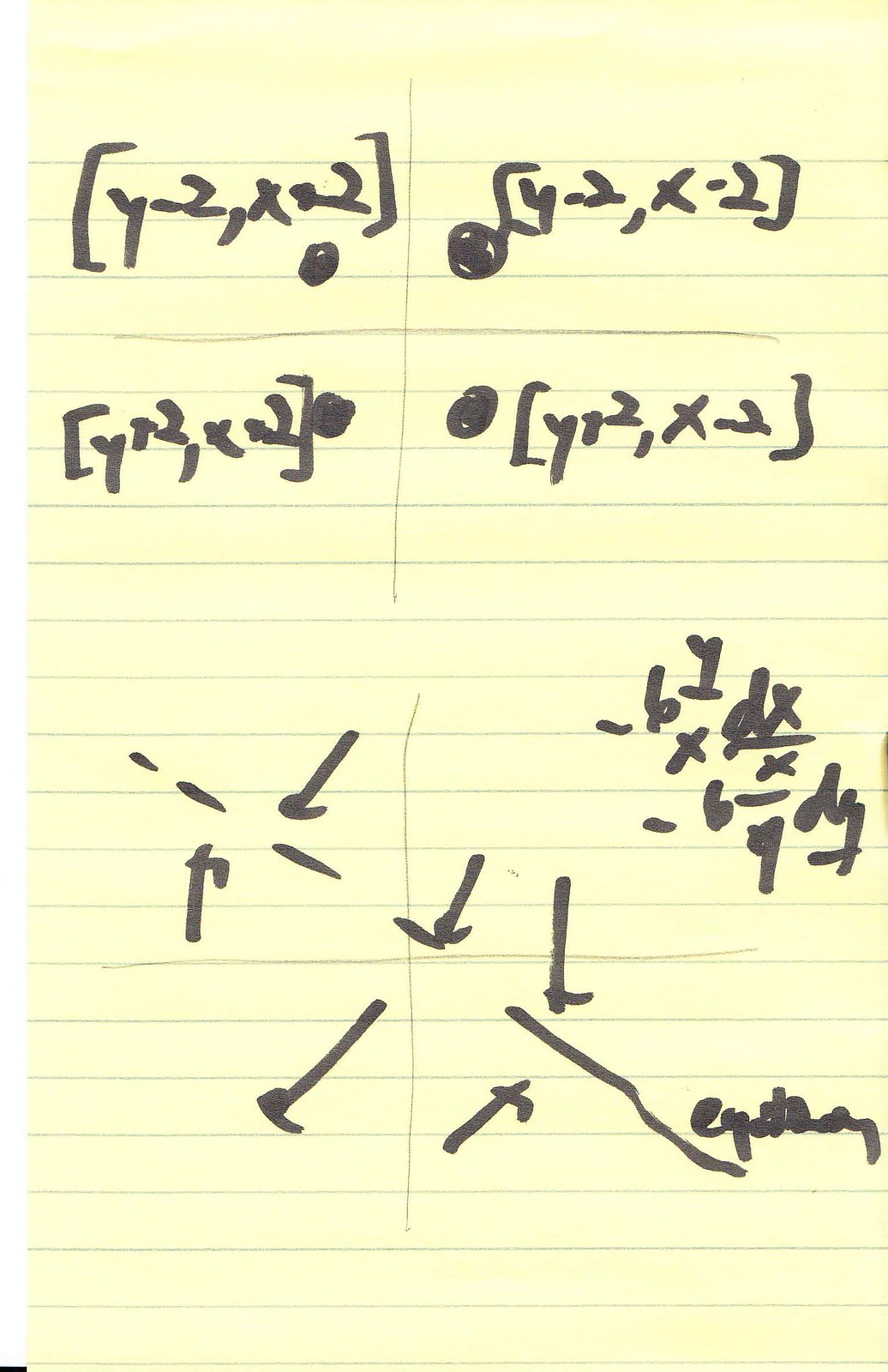An image features a light pink piece of paper with faint lines running through it. There appears to be a delicate vertical line drawn down the center, intersected by a horizontal line about one-third of the way down the page. The sheet is filled with various mathematical notations in black ink. Among these notations are symbols such as Y₂, X₂, a dot underneath, Y - 2, X - 2, Y + 2, 2Y, X - 2, a negative sign, 61, X, and DX over X. Additional expressions like 6, 9 DX are also present. An area of the paper has a pattern of dotted lines and several arrows. Three arrows point downward, two point upward, and another arrow in the middle is oriented somewhat downwards. There is also an indistinguishable word written in black. The overall appearance is of a page filled with calculated figures, graph lines, and directional arrows, all meticulously placed on this small, pink, lined paper.